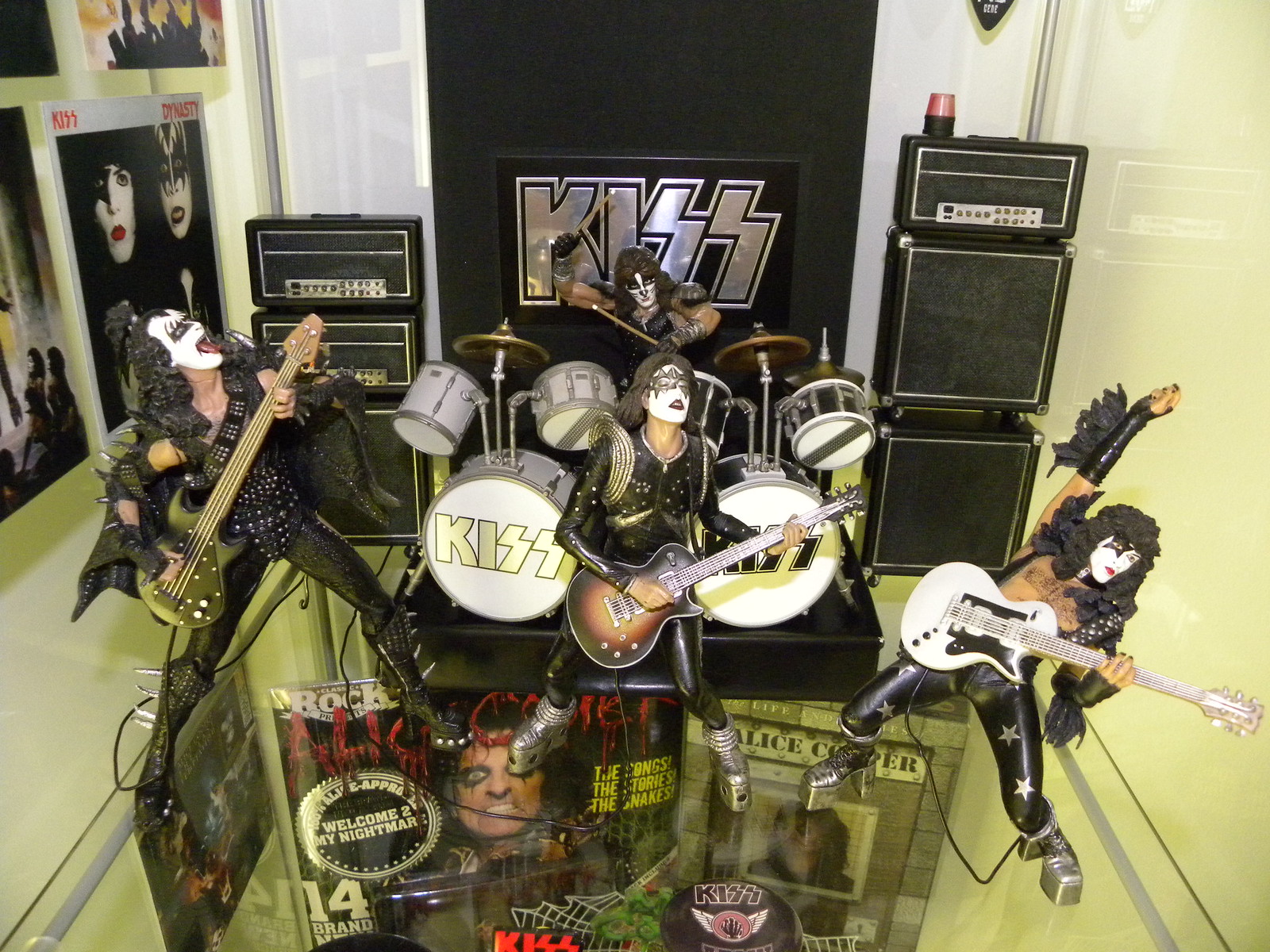This brightly lit photograph features an elaborate display of collectible KISS dolls, meticulously posed as if performing live in concert. Gene Simmons is depicted with his iconic tongue out, amplifying the lifelike dynamism of the scene. The dolls are equipped with their musical instruments and set against a backdrop that includes towering guitar speakers and amplifiers. The KISS logo prominently adorns the drum kit, which is staged at the center of the display. The black panel behind the dolls showcases a chrome-colored KISS logo, enhancing the rock ambiance. Supporting elements such as Alice Cooper merchandise and additional KISS items are visible through the glass shelf beneath the dolls. On the left side of the image, tastefully mounted photographs or album covers add to the display’s authenticity, emphasizing the dedication of a true fan. The entire scene is framed by walls and a floor with a yellowish-gold hue, adding a warm glow to the rock-themed setup.